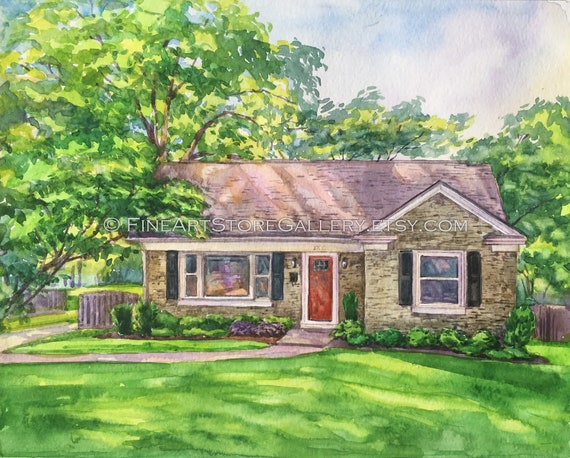This artistic painting, copyrighted by fineartstoregallery.etsy.com, depicts a charming, small one-story house with a blend of realistic and whimsical elements. The house, primarily constructed of light-colored stone or brownish bricks, features a notable hipped roof in shades of gray and black. The front door is a striking red with white trim, flanked by windows adorned with white trims and black shutters. A curving concrete sidewalk leads up to the door, bordered by neatly trimmed green bushes. Surrounding the house is a lush, vividly green lawn extending to a picket fence that's visible on the right side. In the background, trees with brown branches and a mix of dark and bright green leaves provide a natural canopy, blending into a sky with soft blue and white hues, evoking a serene summer day. The image is softly detailed, contributing to its artistic charm.